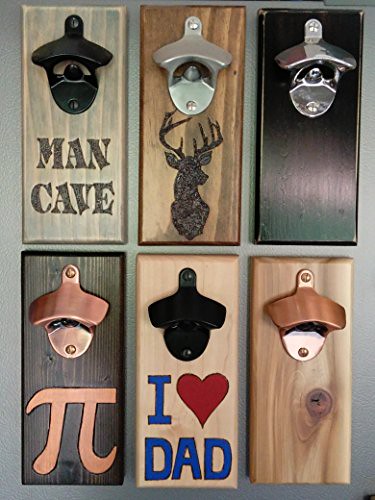This photograph showcases six wooden plaques, each adorned with a distinctive mounted bottle opener. Arranged three on top and three on the bottom against a light gray background, these plaques each present unique designs and textures:

1. The top left plaque has a black bottle opener on a tan and greenish wood background with the words "Man Cave" inscribed underneath.
2. The top middle plaque features a silver opener set against a darker, grainy brown wood with an intricate deer head and antlers design, seemingly burned into the wood.
3. The top right plaque is simple yet elegant, with a polished silver opener mounted on a solid black wooden background.
4. The bottom left plaque is dark brown wood with a copper opener, displaying a black painted pie symbol.
5. The bottom middle plaque is a lighter wood with the phrase "I Love Dad" in blue capital letters and a red heart, complemented by a black opener.
6. The bottom right plaque, made from a sanded-down cedar with a noticeable knot, includes another copper opener and features a symbol that appears to represent Chinese peace.

Each plaque, with its combination of wood type and bottle opener finish, contributes to an intriguing, stylistic variety perfect for a rustic bar or man cave.